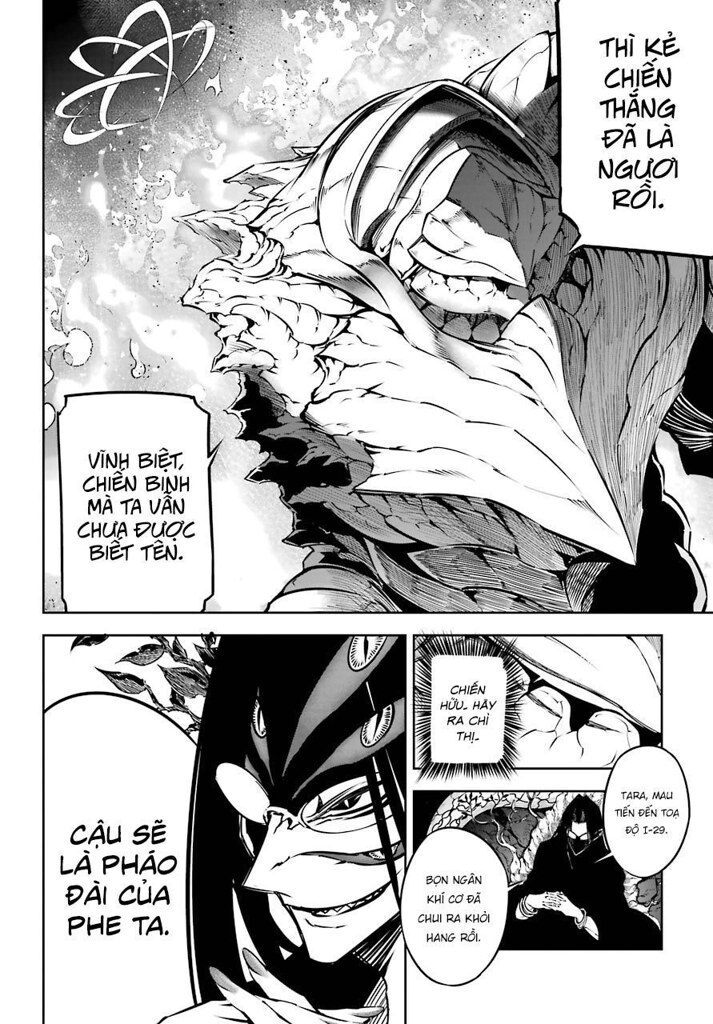The image showcases a black, white, and grey comic strip or comic book page divided into distinct sections, with a high composition and foggy, wet background tones. In the top-left corner, there is an abstract insignia with intertwining streaks of arches. The top section features a large square panel. The character in this panel bears a fantastical, arthropod-like appearance, resembling a sea crab or roly-poly with numerous eyes lacking irises. The speech bubbles, in what appears to be Vietnamese or Chinese, add to the narrative ambiguity.

Below, the comic splits into three smaller panels. The first smaller panel on the bottom left showcases a humanoid character with spider-like design attributes, featuring multiple eyes extending up the skull. This character wears glasses and has slits below human-like eyes. Their hands are folded thoughtfully. In the central smaller panel, the text bubbles suggest dialogue, while the imagery focuses on an abstract close-up of eyes, possibly those of the first character. The bottom smaller panel continues the narrative with additional speech bubbles and a wider shot of the character on the left, maintaining the comic's eerie and complex aesthetic.

Overall, the recurring themes of abstract designs and otherworldly characters create a visually striking and mysterious scene, enriched by detailed speech and thought bubbles in a non-English language.